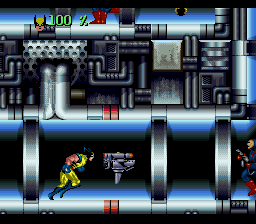This image is a screenshot from an animated video game, likely a mobile game, based on the X-Men franchise. The scene is set in an industrial, factory-like hallway with silver, chrome-looking bars visible in the background, suggesting a high-tech environment. At the very top of the screen, there is a green indicator displaying '100', signifying that the character Wolverine is at full health. Next to this health indicator, there is a small icon of Wolverine's face, easily recognizable by his distinctive yellow hat and black winged helmet. The main focus of the image is Wolverine, who is depicted running toward the right side of the screen. He is dressed in his traditional yellow and blue X-Men outfit, complete with blue boots, yellow pants, blue gloves, and a mask covering his pale skin. The overall image captures a dynamic moment in the game, emphasizing Wolverine's readiness for action in his iconic attire.